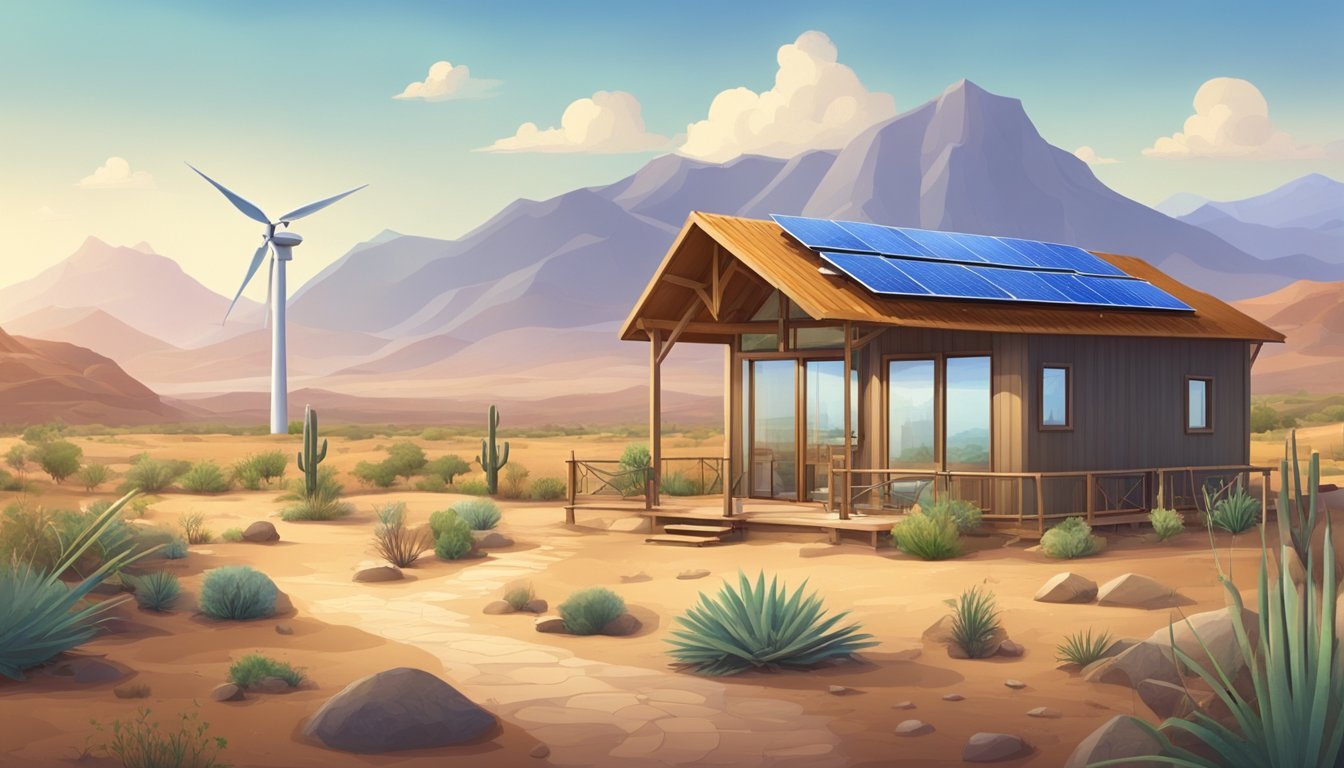This detailed artistic design depicts a small, sustainable house situated in a barren desert landscape. The foreground is a dusty brown dirt path, dotted with various desert plants, like ferns and cacti. To the left, a tall, white wind turbine stands prominently against the backdrop of a blue sky. Desert shrubs and rocks scatter across the scene, providing a stark contrast to the sandy ground. In the background, rugged gray mountains stretch across the horizon beneath the expansive blue sky, which is adorned with five wispy clouds. The focal point of the image is a modest cabin positioned slightly to the right. The house features double glass doors at the front, leading to a wooden porch. Its roof is fitted with blue solar panels, emphasizing the sustainable theme. The overall color palette consists of warm shades of orange and brown, hinting at a sunset ambiance that adds a serene touch to this envisioned eco-friendly desert abode.